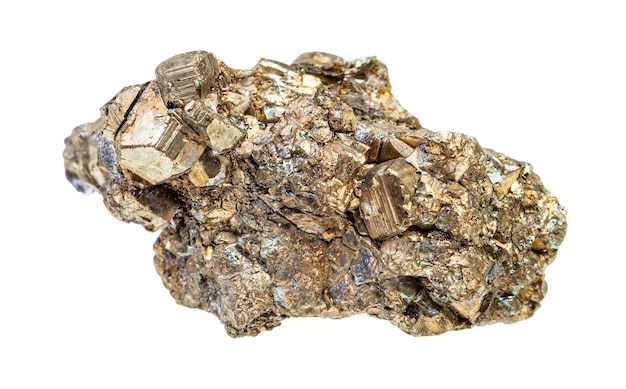This image showcases a highly textured, golden mineral nugget, prominently set against a stark white backdrop. The rock, positioned centrally, boasts a striking variety of colors including bright gold, bronze, dark gray, and hints of silver. Its ovular shape is characterized by numerous indents, crevices, and crevasses, with the middle part appearing larger and more rounded compared to its relatively pointy ends. The intricate surface reflects light brilliantly, emphasizing its potential value and metallic nature. Despite the uncertainty of whether it is purely gold or another type of mineral, the detailed, fragmented structure and diverse coloration highlight its unique and precious qualities.